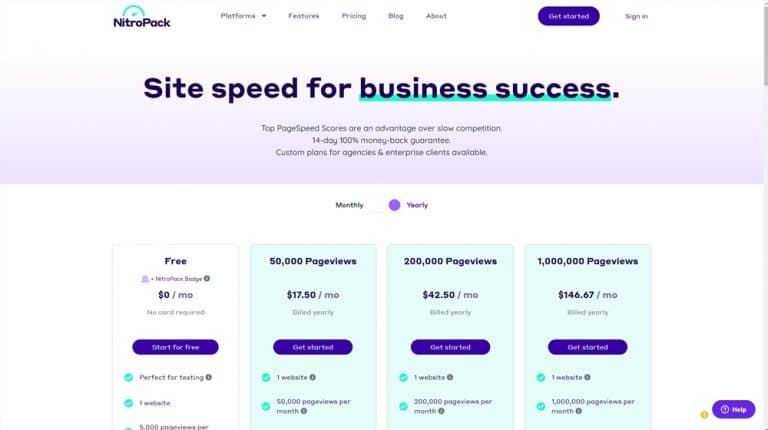The top part of the image features an ombre background that transitions from white to light purple. On the left-hand side, the text "Nitro Pack" is displayed in purple, although it gets a bit blurry in some sections.

The navigation menu across the top includes tabs labeled "Platforms," "Feature," "Price," and "Blog About." Next to these tabs, there's a purple button with white text that reads "Get Started," followed by another link in purple or black that says "Sign In."

Centrally located on the page, a bold purple headline announces "Site Speed for Business Success," with the phrase "Business Success" underlined in teal and followed by a period. Below this headline is a smaller font paragraph that's harder to read, stating, "Top page speed scores are an advantage over slow competition. 14-day, 100% money-back guarantee. Custom plans for agency enterprise clients are available."

Towards the bottom of the image, there are four pricing rectangles. The first rectangle, with a white background, is labeled "Free" and priced at "$0/month," suitable for testing one website with 5,000 page views per month, although the text gets cut off. The next three rectangles have teal backgrounds. The second rectangle offers 50,000 page views and is priced at $17.50 per month. The third rectangle allows for 200,000 page views at a price of $42.50 per month. The fourth and final rectangle accommodates one million page views, priced at $146.67 per month.

Each of these three teal rectangles features a purple oval button with white text that reads "Get Started."